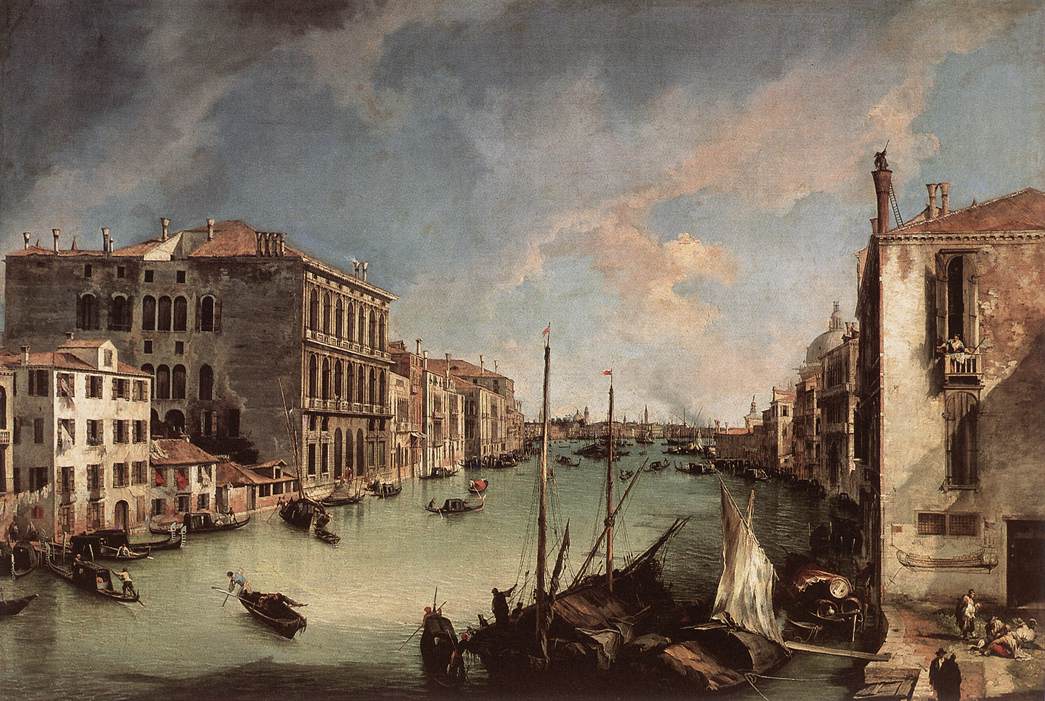The painting depicts a bustling scene along one of the main waterways of Venice, Italy. The long, rectangular artwork is richly detailed, showcasing a balance of daily life and intricate architecture. On the left side of the painting, several gondolas are seen departing and arriving, indicating a hub where gondoliers either pick up customers or take breaks. A couple of private vessels for merchants or fishermen also feature prominently, with a handmade wooden walkway connecting the boats to the buildings.

To the right, various ships with sails at different stages of being raised or lowered add to the dynamic nature of the scene. A tattered, makeshift boat with worn white sails sits near a group of people, lending a sense of authenticity and lived-in charm. The buildings on this side are equally captivating – one features an old woman peeking out from a small veranda on the second floor, while another has a man diligently cleaning a chimney on the rooftop. The windows of the buildings are open, inviting the moody, overcast sky into the composition.

The artist’s meticulous attention to detail is evident in the realistic fine lines, suggesting the use of ink before applying paint. The background seamlessly illustrates gondolas weaving through the waterway, enhancing the liveliness of Venice’s timeless allure.